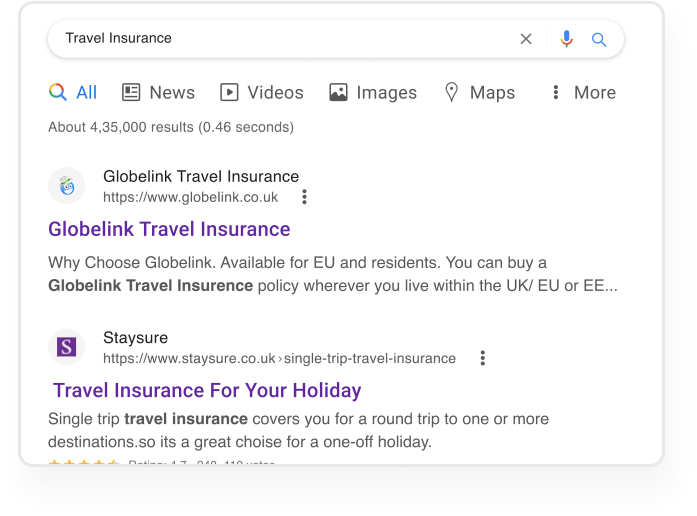**Descriptive Caption:**

The image captures a partial Google search results page for "travel insurance" as viewed on a smartphone. At the top of the screen, the search box contains the phrase "travel insurance," followed by a close icon, a Google microphone icon, and a search icon. Right below the search bar, Google's navigation tabs are displayed, showing "All" as the active tab, with additional tabs for "News," "Videos," "Images," "Maps," and a "More" option represented by three vertical dots.

The search results indicate around 4,035,000 results delivered in 0.46 seconds. The first highlighted result is from "GlobalLink Travel Insurance" with the URL GlobalLink.co.uk. The link has already been clicked, and the summary reads: "GlobalLink travel insurance. Why choose GlobalLink? Available for EU and residents. You can buy a GlobalLink travel insurance policy wherever you live within the UK/EU/EE."

The second result is from "Staysure" found at Staysure.co.uk, with a URL path suggesting a single trip travel insurance plan. The description for this result states: "Travel insurance for your holiday. Single trip travel insurance covers your round trip for one or more destinations, making it a great choice for a one-off holiday."